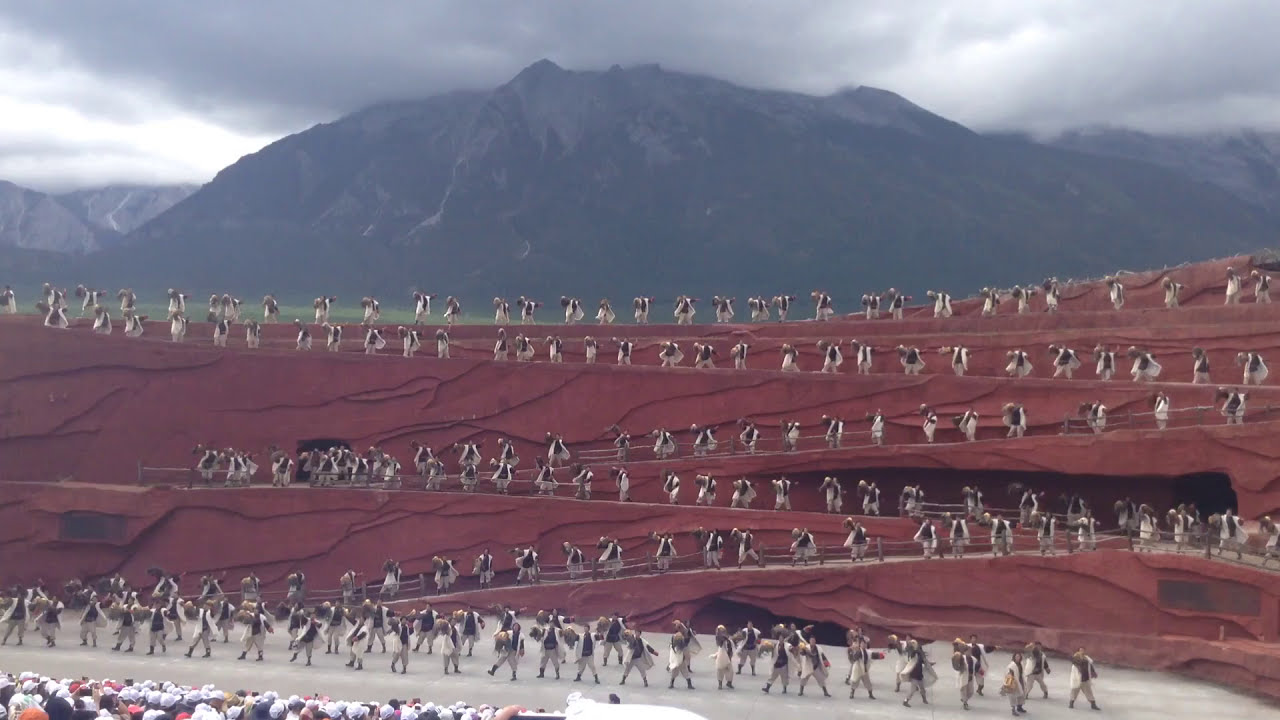The image depicts a dramatic scene featuring a colossal mountain range in the background with dark gray and light gray skies, possibly at dusk. In the foreground, there's an imposing maroon rock formation with a sandy, almost man-made appearance, criss-crossed by a network of zigzagging pathways. These pathways, numbering about seven levels, are occupied by numerous figures dressed in similar uniforms, featuring large white coats and hard white hats that suggest they might be involved in a performance or celebration rather than construction work. The rock structure includes several black openings resembling caves. At the very base, there's a white, rocky ground with a flat road, where some additional figures can be seen standing or sitting. The entire scene is awash with an atmosphere that combines natural grandeur with human activity, possibly set against a snowy mountain backdrop that highlights the outdoor setting. The presence of clouds adds to the impression of a bustling yet serene midday moment.